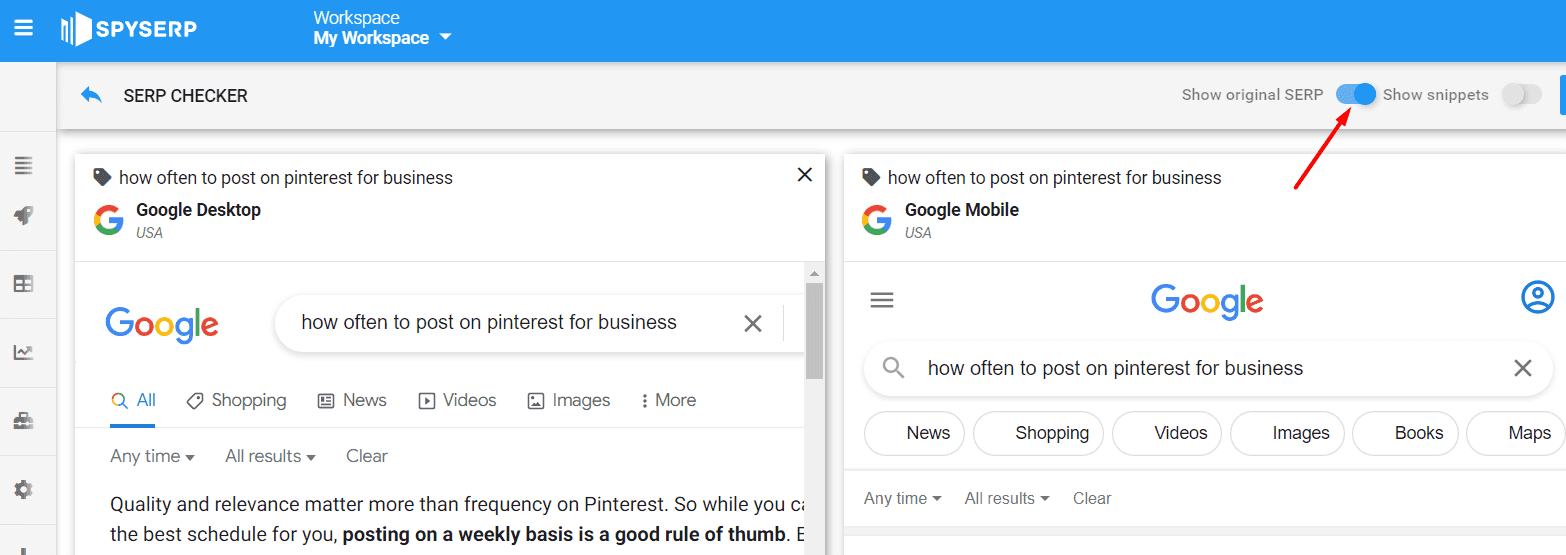The image is a screenshot of a website that features a blue banner at the top with the text "Spy SERP." To the left of the text is a logo resembling white books. To the right of this, there is a dropdown menu labeled "Workspace" followed by "My Workspace." Below the banner, in black text, it says "SERP Checker." 

Underneath, there's a search query displayed: "How often to post on Pinterest for business." Alongside this search query, the Google logo and the text "Google desktop USA" are visible, indicating that the search is being conducted on Google. The search bar contains the text: "How often to post on Pinterest for business." The subsequent informative text within the search bar mentions, "Quality and relevance matter more than frequency on Pinterest. So while you the best schedule for you, posting on a weekly basis is a good rule of thumb."

To the right of this main search query is an alternative suggestion for the same query. Below all this, the interface displays buttons for different search categories: "News," "Shopping," "Videos," "Images," "Books," and "Maps."